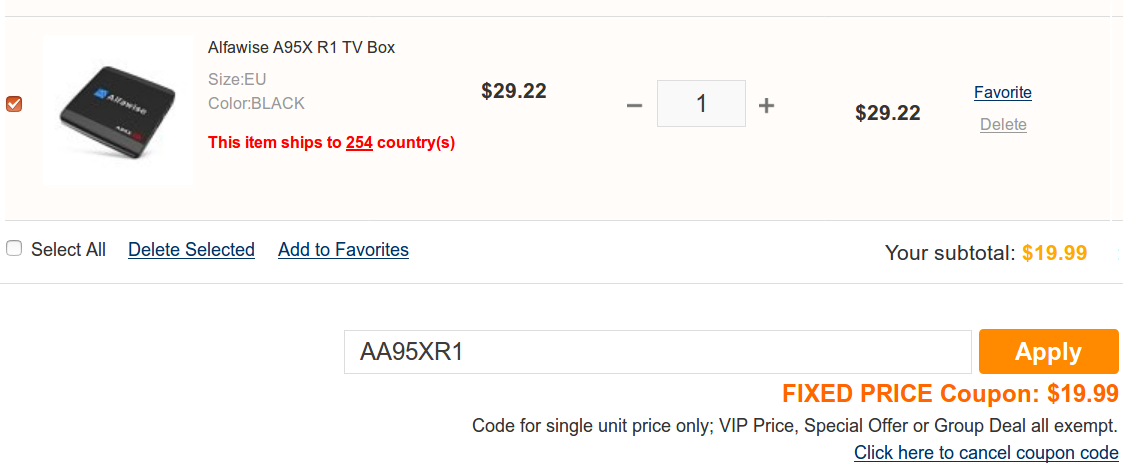Screenshot of a user's shopping cart from an undisclosed e-commerce website. The top of the cart displays an orange checkmark indicating the validity of the items listed. Below the checkmark is an image of the item being purchased: an Alfawise A95X R1 TV box, size EU, in black color. In red text beneath the image, it states that this item ships to 254 countries. The item is priced at $29.22, and the user has selected one unit, making the subtotal $29.22. 

Next to the item, there are links to mark it as a favorite or to delete it from the cart. Below the itemized section, options are available to select all items in the cart with a corresponding checkbox, and buttons to either delete the selected items or add them to favorites. 

The subtotal displayed at the bottom of the cart is $19.99, indicating that a coupon code 'AA95XR1' has been applied. This coupon offers a fixed discount, reducing the price to $19.99. There's a note clarifying that the coupon is only applicable for a single unit at its standard price, and cannot be used in conjunction with VIP prices, special offers, or group deals. A link is provided to cancel the applied coupon code if needed.